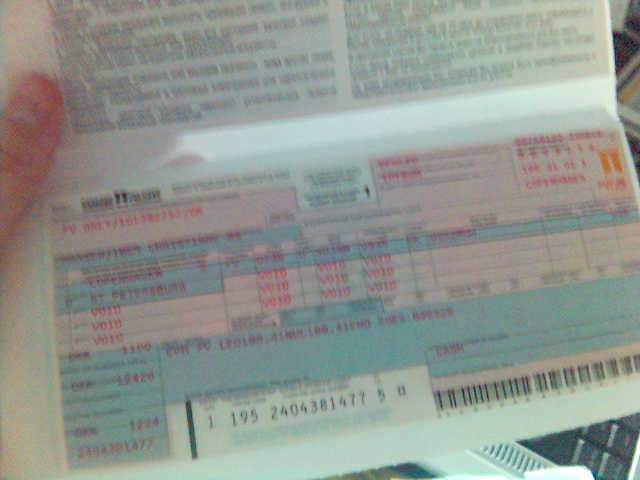The image depicts a blurred printout resembling the interior of a checkbook-sized receipt. Dominating the printout are multiple instances of the word "void," indicating previously voided transactions. In the upper left corner, there's a logo that likely represents a financial institution. The lower right section of the image features a barcode and part of a computer keyboard. At the very bottom, a string of numbers (1-195-2404-381-4775) appears, which could be associated with account details, a routing number, or a check number. Despite the blurriness, the printout seems to be a record of past financial transactions that have been voided.